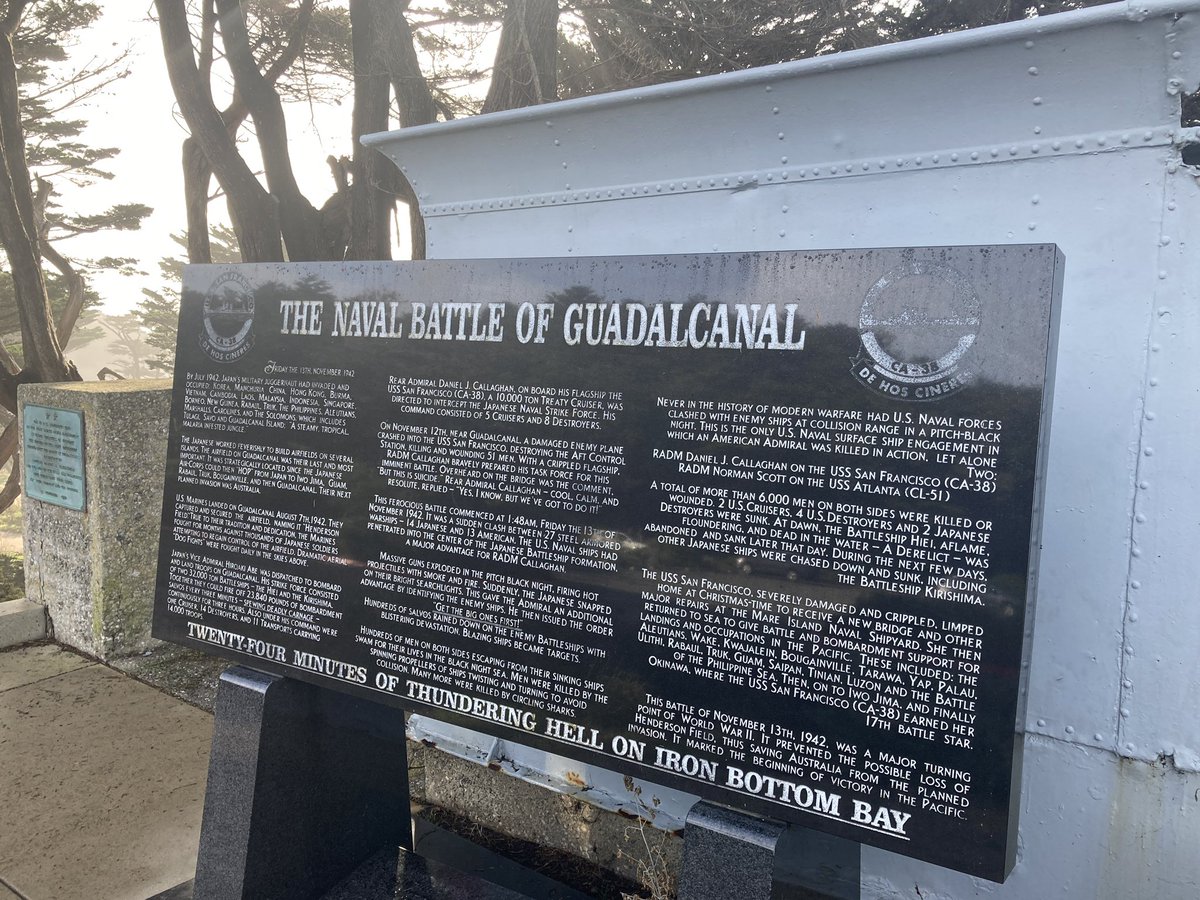The image captures a historical marker commemorating the Naval Battle of Guadalcanal, a significant World War II conflict in the South Pacific. The foreground features a prominently black plaque with white text, detailing the battle across 14 small paragraphs. At the bottom of the plaque, bold text declares, "24 minutes of thundering hell on Ironbottom Bay." This plaque stands on a riveted pedestal made of light blue metal, situated on a cement area. The background reveals a serene woodland setting with large mature trees bathed in midday sunlight, under a cloudy sky. The scene appears to be part of an outdoor memorial site dedicated to this pivotal naval engagement, inviting visitors to explore and reflect on its historical significance. Two emblems adorn the plaque, with the right-hand emblem labeled CA-3B, possibly associated with the ship Dejo Cenere.